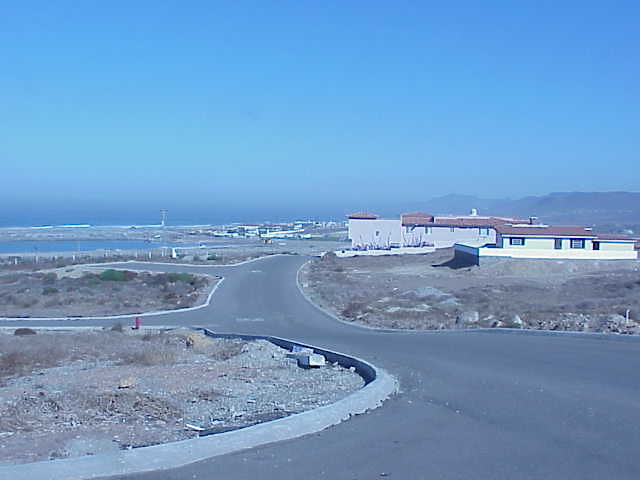The image captures a quiet, seemingly desolate new housing development on the outskirts of some town. A paved road winds through the scene, bordered by roundabouts scattered with dust, tumbleweeds, sand, and grass. Dominating the right side is a one-story, light gray house with a brown roof, perched on a small hill. The house's windows catch the light, set against a vivid blue, cloudless sky that stretches expansively above.

In the background, serene waters—possibly a large lake or the ocean—can be seen, with the faint outlines of a small town and additional homes that are in various stages of completion. This new development appears close to nature, as there are mountain ranges visible in the right-hand corner of the image, adding a rugged backdrop to the otherwise tranquil scene. The overall atmosphere is quiet and empty, devoid of people, animals, or any evident activity, lending an almost surreal quality to the landscape.